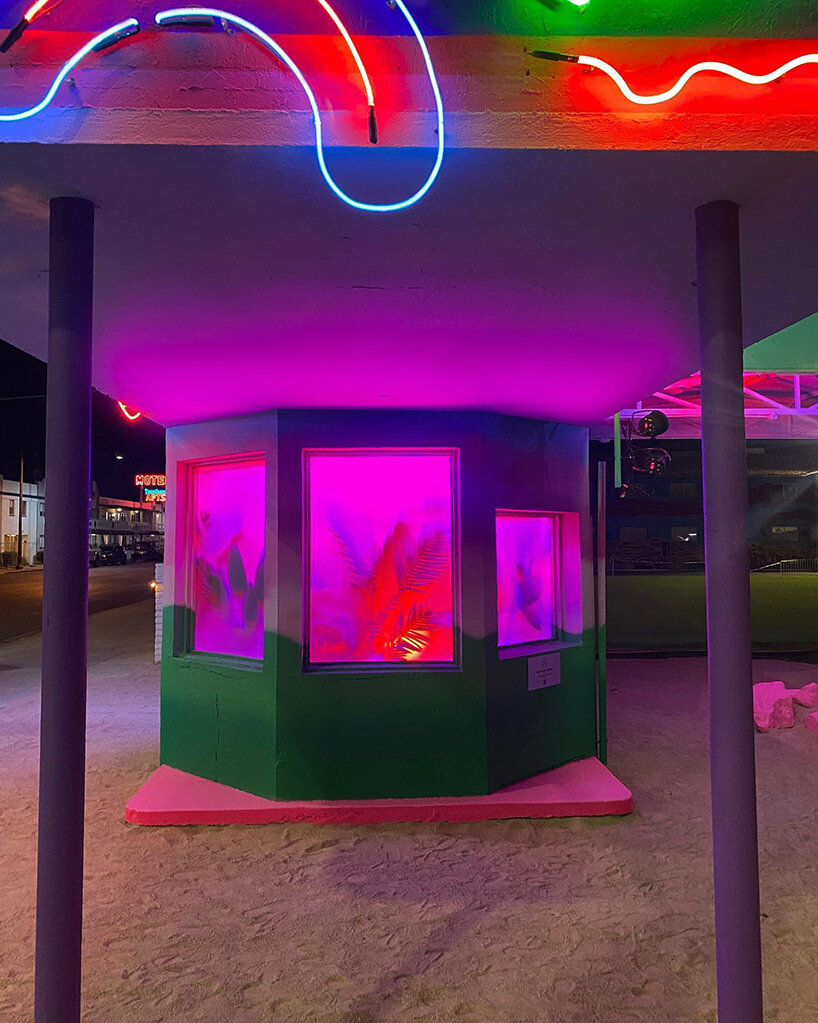The photograph captures an outdoor scene with a sandy ground and a small, intriguing structure. In the foreground, two purple posts support a flat, covered roof adorned with vibrant neon signs. One sign, on the top left, has a distinct shape, while the other, on the top right, features a squiggly design. Beneath the roof, there's a green-walled, blocky, octagonal building that transitions into purple towards the top. It rests on a thick red base. The building has several windows with a purple tint through which you can see illuminated plants. The structure emits an ambient purple light, adding to the neon glow. The setting is reminiscent of a fairground with various buildings in the background.